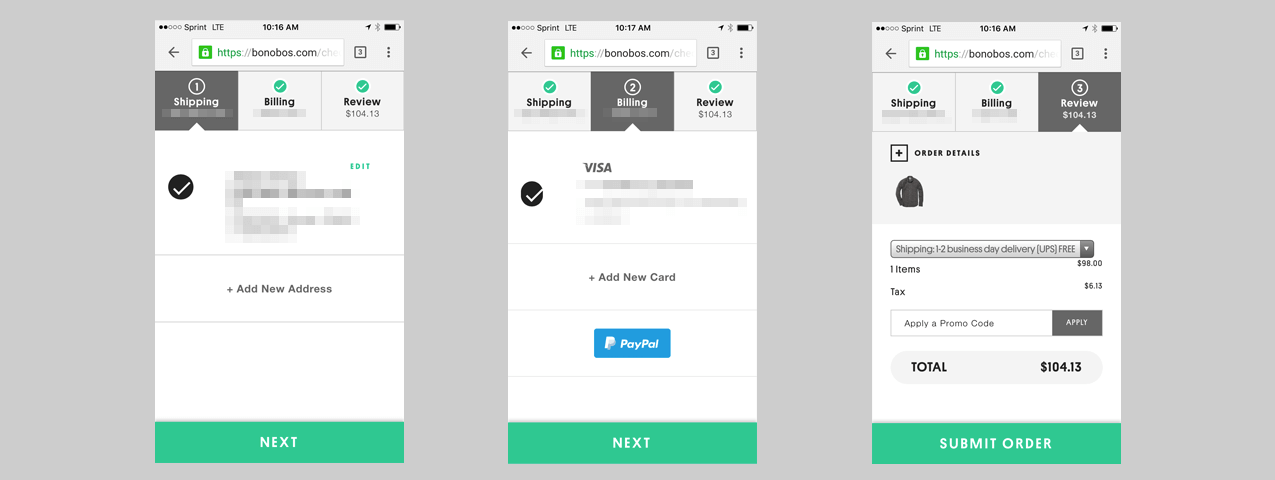This image is a screenshot displaying three distinct order pages from Bonobos.com, arranged side by side against a gray background.

1. **Step One: Shipping** - The leftmost section is labeled "Step One: Shipping." Below this title, there is a blurred-out product item with an adjacent checkbox for selection. Further down, there's the option to "Add New Address," followed by a prominent green rectangular button labeled "Next Step."

2. **Step Two: Billing** - The center section is labeled "Step Two: Billing." It shows grayed-out card information, specifying that the entered card is a Visa. Beneath this, there is a blue button featuring the PayPal logo and the option to pay with PayPal. The section concludes with a repeated green button, also labeled "Next Step."

3. **Step Three: Review** - The rightmost section is labeled "Step Three: Review" and displays the order total of $104.13. Below this, there's a square box with a plus sign for order details, including a small thumbnail image of a jacket. A dropdown menu for shipping options is visible, with "1 to 2 Business Day Delivery" selected. The pricing details are broken down as follows: one item totaling $98, with an additional tax of $6.13. There's an option to apply a promo code with an adjacent button labeled "Apply." At the bottom, an oval-shaped gray box reiterates the total amount of $104.13, followed by a green button labeled "Submit Order."